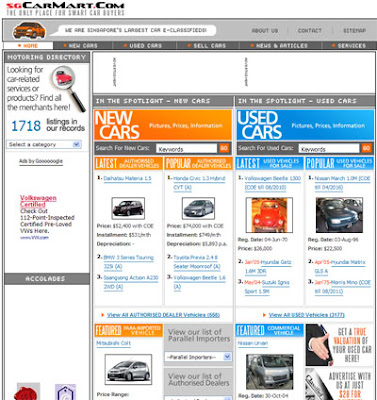The screenshot appears to be from the website sgcarmart.com, which is branded as "the only place for smart car buyers." In the upper left corner, the website’s logo is prominently displayed along with its slogan. Below this, there is an image of a small orange car.

The main section is divided into categories starting with "New Cars," highlighted by an orange background. This section includes a search bar to help users find specific vehicles. Directly beneath are subsections labeled "Latest New Cars" and "Popular New Cars," where users can click on various car listings to view detailed prices and information.

Adjacent to this is a blue rectangle that indicates the "Used Cars" section, also featuring a search bar. Below this, there are small rectangles with a white background displaying images of used cars. To the left, a red Volkswagen stands out, reminiscent of an older model, while to the right, there is a blue sedan.

Further down the page, two featured cars are showcased: one is a new gray van, and the other is a used gray van, giving prospective buyers an insight into the range of options available.